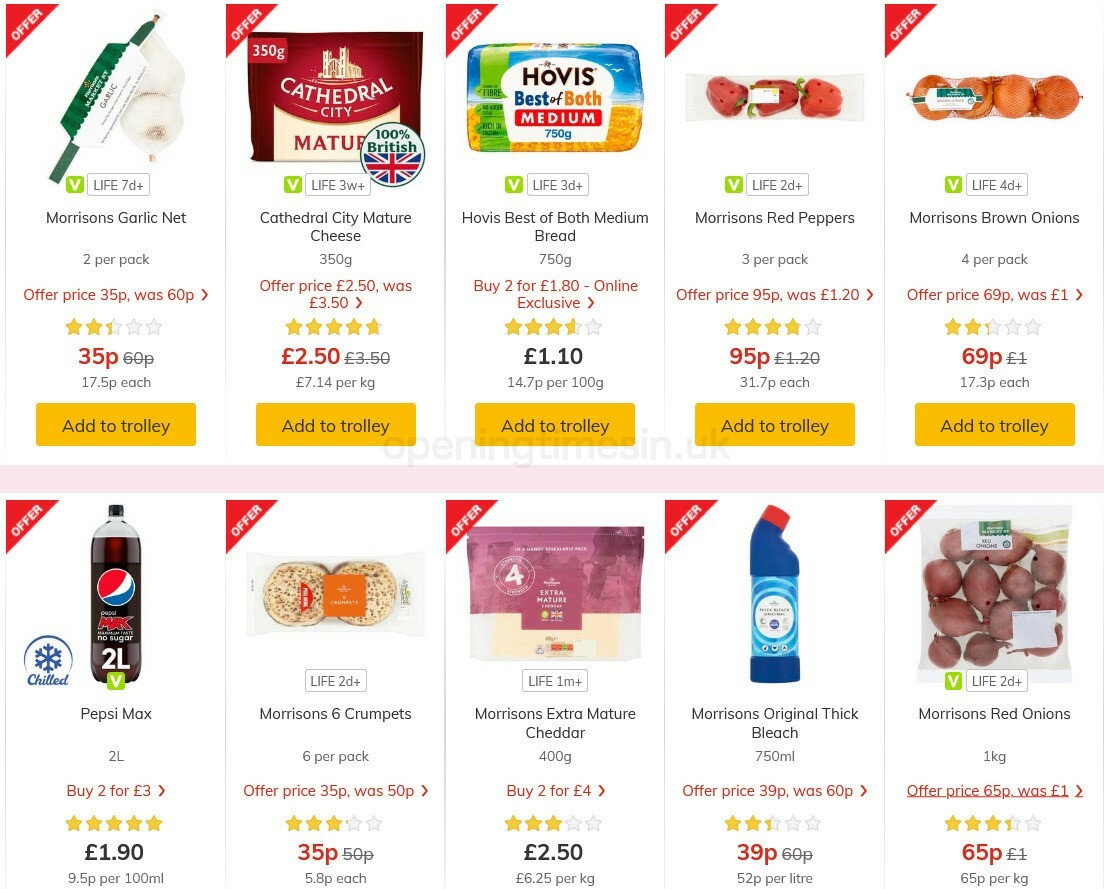This shopping page from a supermarket features a grid layout with two rows of five squares each, showcasing a variety of purchasable items. Each square contains a detailed photo of the product, a corresponding description, an offer price, and a convenient 'Add to Trolley' button.

In the first row:
1. The first square displays "Morrison's Garlic Net" with an image of fresh garlic heads wrapped in a net.
2. The second square features "Cathedral City Mature Cheese," depicting the product's label adorned with a badge proclaiming "100% British" alongside a British flag.
3. The third square presents "Hovis Best of Both Medium Bread," showing the brand's recognizable packaging.
4. The fourth square offers "Morrison's Red Peppers," illustrated by a photograph of three vibrant red peppers neatly wrapped in cellophane.
5. The fifth square showcases "Morrison's Brown Onions," featuring a package of four hearty onions.

Each item is meticulously described so shoppers can easily identify and purchase the products they need.